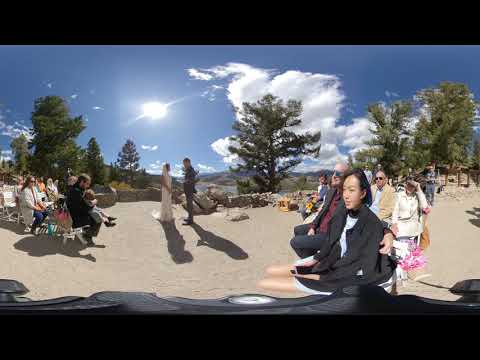This digital photograph captures an outdoor wedding set against the backdrop of a serene, sandy beach area. Dominated by a sunny sky with a few fluffy clouds, the image features a solid black border along the top and bottom edges. At the center, the bride dressed in white and the groom in dark attire stand facing each other, enveloped by a large group of over a dozen attendees. Some spectators are seated on the left-hand side on chairs, attentively facing the couple, while others on the right seem distracted, gazing towards the left across the scene. The setting, possibly a public park, is accented with scattered trees and mountains in the background, bathed in the midday light. The image is rich in colors: black, blue, white, grey, green, orange, pink, maroon, and yellow, giving a vibrant, lively feel to the celebratory moment. No text is visible in the image.